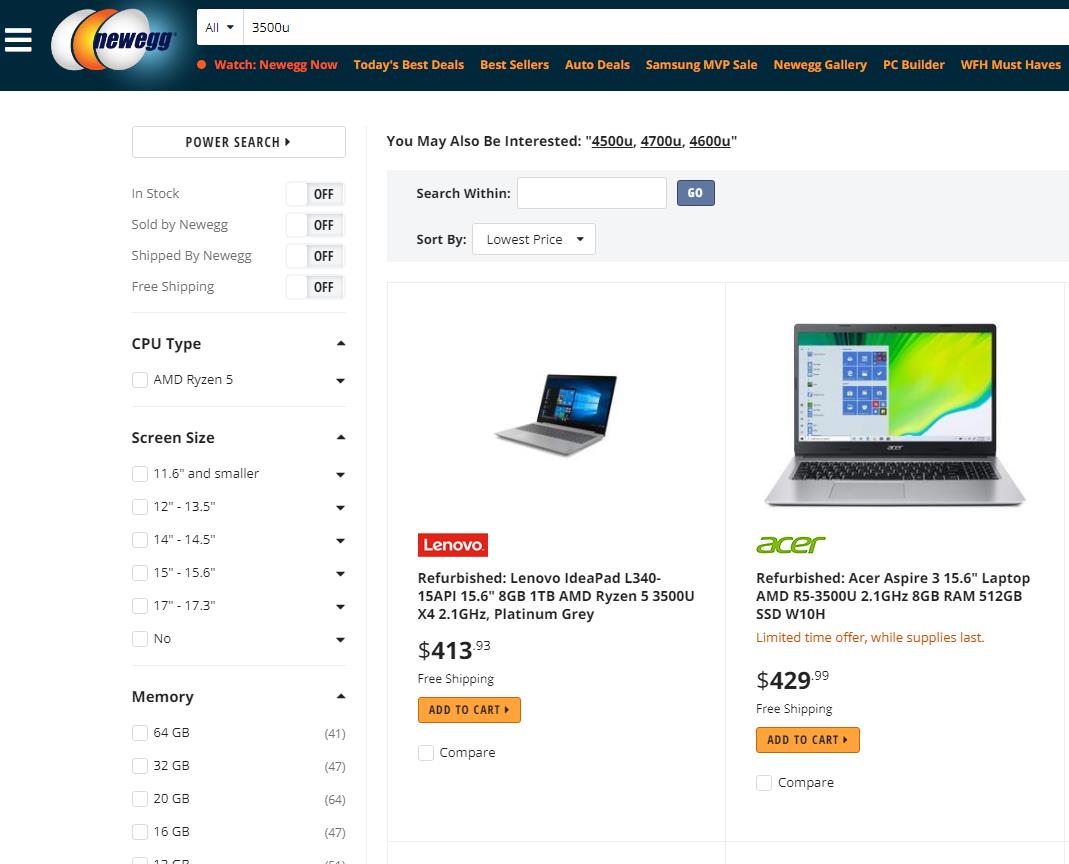This image is a detailed screenshot from the Newegg website's computer section. At the very top, a black banner spans the width of the page. On the top left corner of the banner, there are three horizontal lines representing the menu icon. Next to it, you'll find the Newegg logo. On the right-hand side of the banner is a search bar designed to help users find specific items on the website.

Directly beneath the banner, there's a navigation bar featuring lightly written tabs, making them hard to read. These tabs, written in yellow text, include options like "Today's Best Deal," "Best Sellers," "Auto Deals," "Samsung EVP Sale," "Newegg Gallery," "PC Builder," and "WFH Must Haves."

Situated below these tabs is another, more compact search bar labeled "Power Search." Adjacent to this search bar, there's a prompt saying, "You May Also Be Interested," followed by a list of processor models: 44500U, 4700U, and 4600U.

On the left side of the page, there is a filtering section where users can refine their search by selecting criteria such as CPU type, screen size, and memory.

In the center and extending towards the right are the search results. The first result is a refurbished Lenovo laptop priced at $413.99. This gray Lenovo laptop is positioned at an angle, facing towards the right-hand side, and is listed as the Lenovo ID Pad L346. 

Adjacent to the Lenovo listing is a larger image of a silver Acer laptop. This refurbished Acer Aspire, featuring a 15.6-inch screen and black keyboard, is facing the viewer directly. The Acer logo is displayed below the image in green text, and the laptop is priced at $429.99.